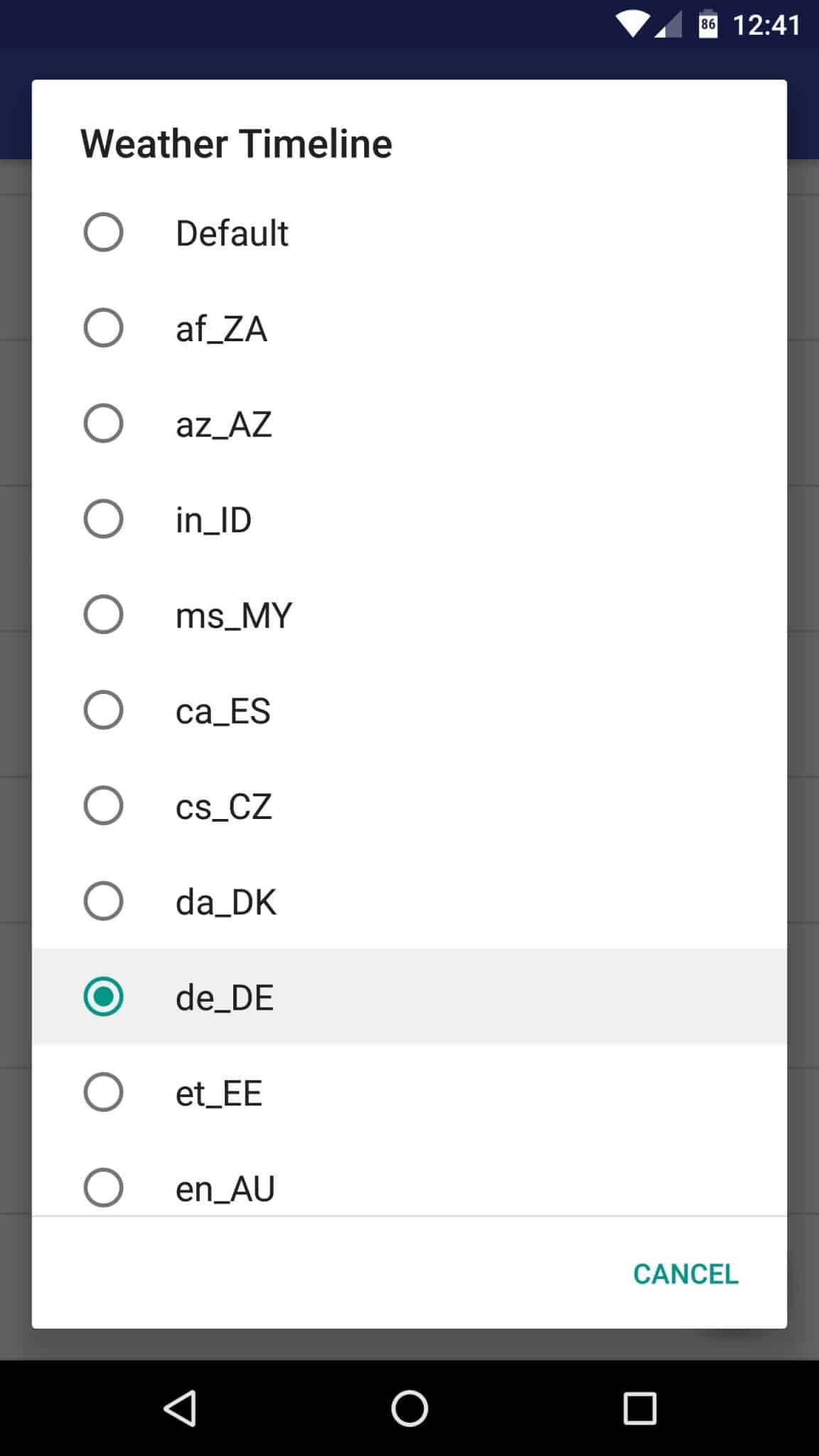This image features the mobile interface of the Weather Timeline application, specifically displaying the language or locale selection menu. At the top, the title "Weather Timeline" is prominently displayed. Below it is a comprehensive list of language or locale options. The options are displayed with their respective codes, such as "default," "af_ZA," "az_AZ," "in_IN," "ms_MY," "ca_ES," "cs_CZ," "da_DK," "de_DE" (selected), "et_EE," and "en_AU." 

Each option is accompanied by a circular selection button on its left side. The currently selected locale, "de_DE," is marked with a blue-green checkmark in its circular button. The interface is designed with a clean and minimalist aesthetic, featuring a white background and black text for easy readability. At the very bottom, there is a green "Cancel" button situated in the right corner.

Additionally, the screen displays the current time as "12:41" and shows an LTE signal with 86% battery strength. The entire list of language options is presented in a scrollable format, ensuring all choices are accessible. The overall interface is straightforward, focusing on functionality and ease of use.